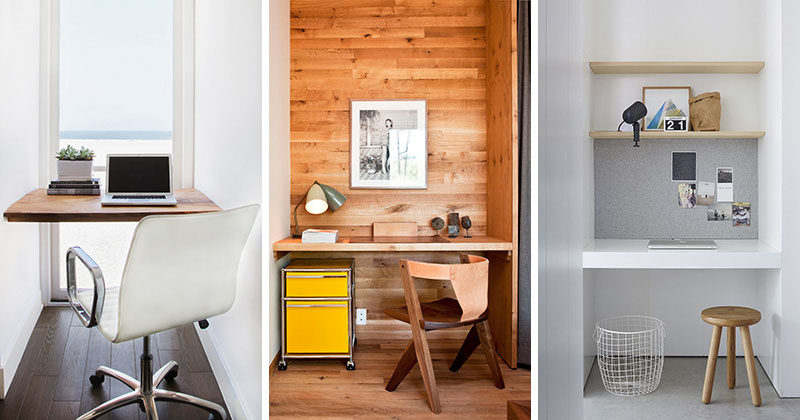The image is a composite of three vertically rectangular photographs, each showcasing a distinct workspace nook within a house. The first photograph on the left features a bright, minimalist office space. It has white walls and a large window that spans across one entire wall, offering a view of a beach or desert scene. A wooden desk sits in front of the window, adorned with a laptop, a planter, and a couple of books. A sleek, white office chair with chrome armrests and wheels completes this serene workspace.

The middle photograph presents a cozy study area with rustic wooden walls and flooring. The desk, also wooden, is fixed between two walls and supported by a yellow file cabinet on wheels. Various objects, including books, are scattered on the desk. A black-and-white photo hangs on the wall, and in front of the desk is a leather-backed chair, adding to the comfortable, lived-in feel of this space.

The third photograph displays a clean, white workspace nook. This minimalistic area features a wooden stool in front of a white desk, which stretches between two white walls. Above the desk, two brown wooden shelves provide additional storage, and a wire trash can sits below. The gray flooring contrasts subtly with the predominantly white decor, while a bulletin board above the desk offers a practical touch.